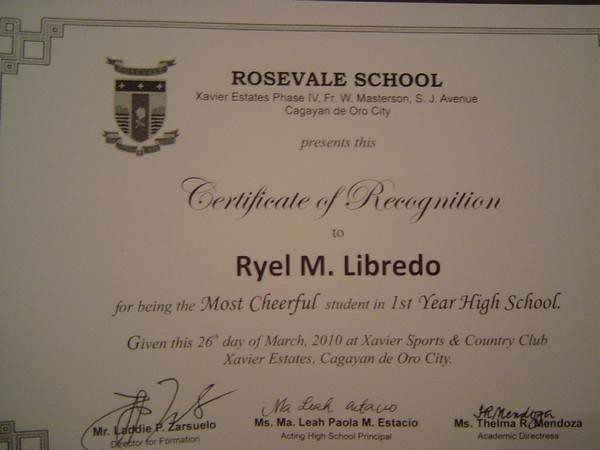This is a landscape-oriented photograph of a Certificate of Recognition from Rosevale Space School. The certificate is printed on an off-white sheet of paper and features a decorative gray border. In the upper left-hand corner, there is a black and gray SHIELD logo, adjacent to which, in bold black uppercase letters, it reads "Rosevale Space School." Beneath that, the address is provided in finer print: "Xavier Estates Phase 4 FRW Masterson, S.J. Avenue," followed by "CAGAYAN DE ORO C."

The certificate prominently displays the text "Presents a Certificate of Recognition" in a black script typeface. Below this, in large black letters, it is awarded to "RYEL M. LIBREDO" for being the "Most Cheerful Student in First-Year High School," with "First-Year High School" and "Most Cheerful" emphasized in bold.

The certificate notes that it was "Given this 26th day of March 2010 at Xavier Sports and Country Club, Xavier Estates, Cagayan de Oro City." At the bottom of the certificate, there are four signatures from various staff members, each with their names typed out below their respective signatures.